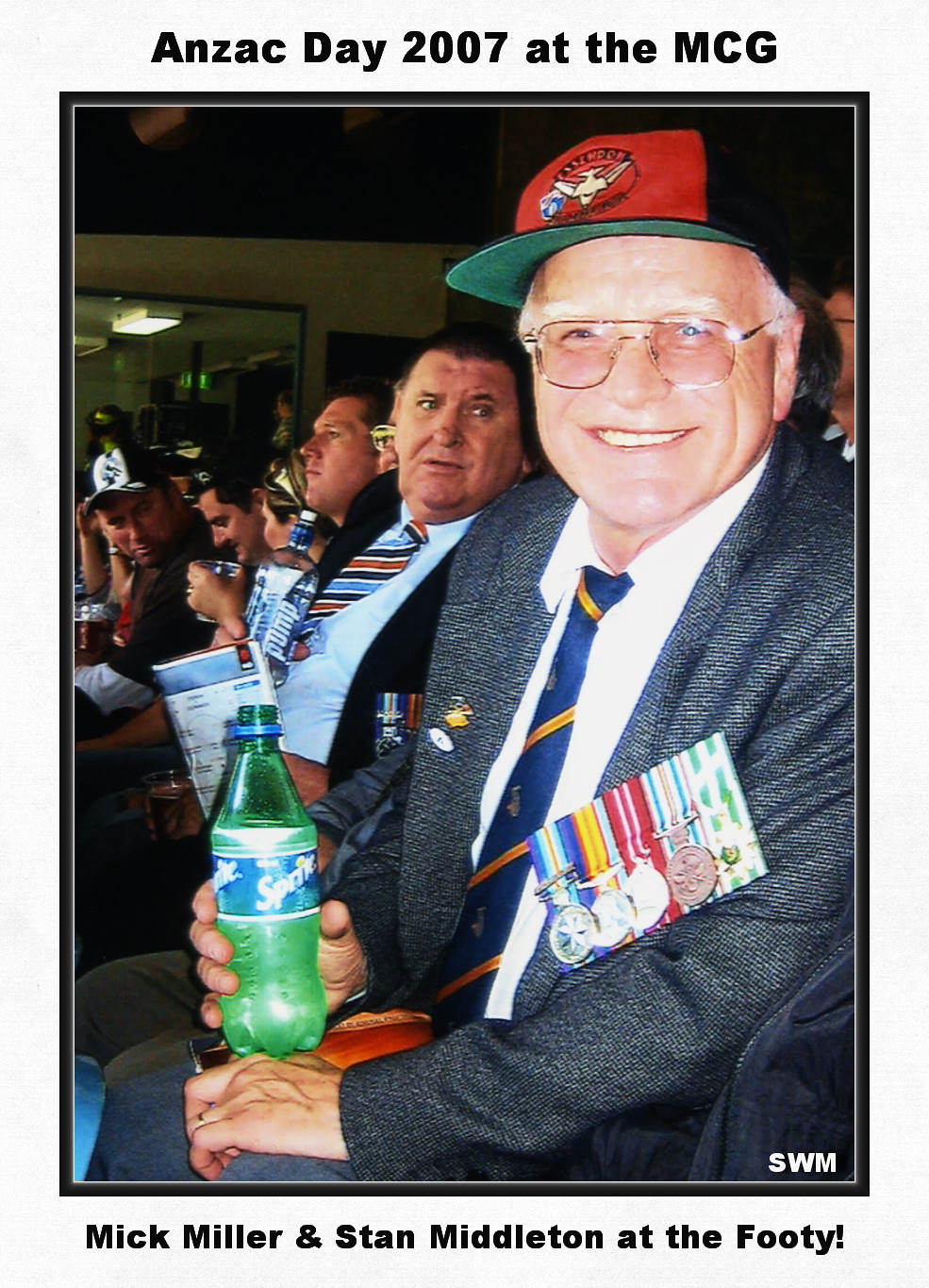The photograph captures a joyful moment among a group of men, predominantly middle-aged and likely of European descent, seated in close proximity. The focal point is an older white male sitting at the front, wearing a red and black baseball cap emblazoned with a symbol. His face is adorned with aviator-style eyeglasses, and he has a broad smile directed at the camera. He is attired in a gray suit complemented by a vibrant blue tie with gold-yellow stripes, and on his left chest, several military medals are proudly displayed. His right hand clutches a green Sprite bottle, appearing freshly opened and invoking a sense of casual enjoyment. Next to him sits another man in a black suit, sporting a tie colored in black, red, and blue. A few seats down, additional men are seen, also dressed in suits and some holding beverages. The photograph frame is white, with the top text reading "Anzac Day 2007 at the MCG," and the bottom text stating "Mick Miller and Stan Middleton at the footy."